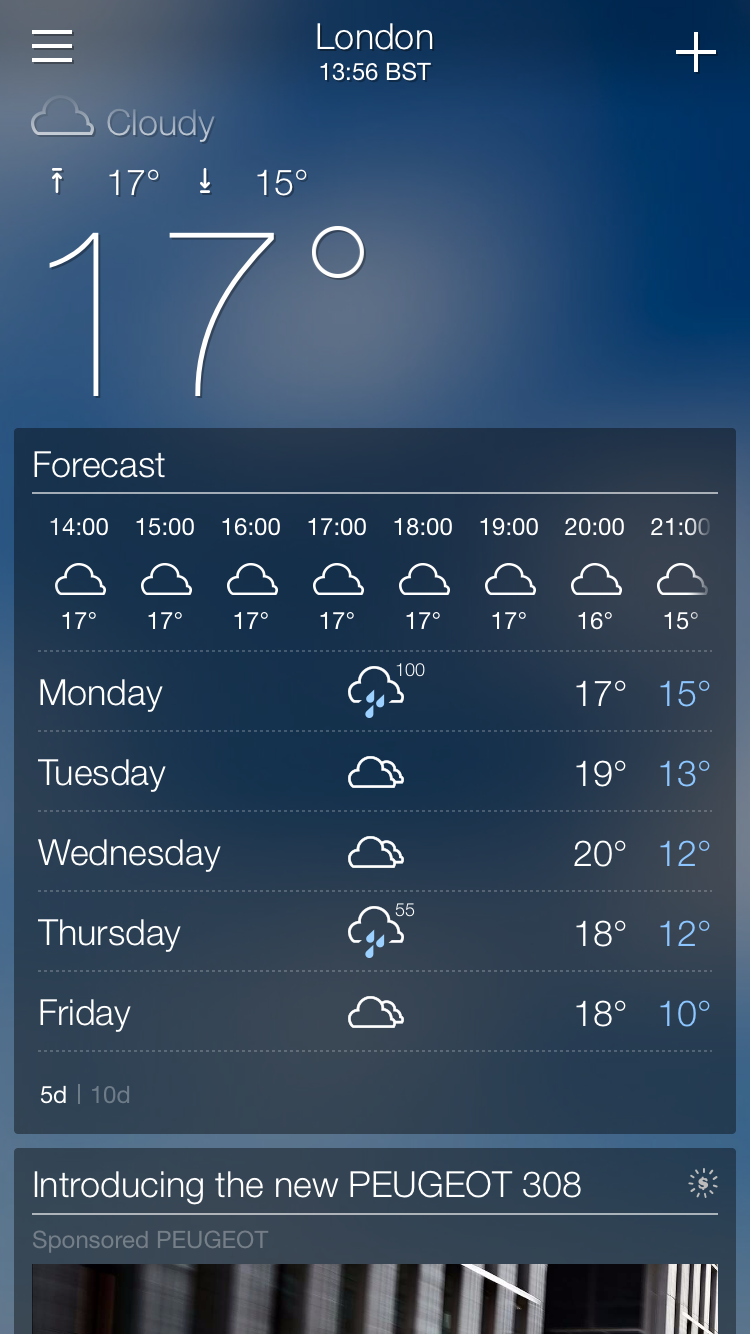A detailed screenshot of a weather app on a smartphone displays the weather forecast for London. The background features a navy blue gradient with a subtle white ombre effect. The displayed time is 13:56 BST. The current weather is noted as cloudy, with the temperature consistently at 17°C. The temperature for the rest of the day remains steady at 17°C through 18:00, drops to 16°C at 20:00, and further declines to 15°C at 21:00, all indicated with a cloudy icon.

The hourly forecast shows the following:
- 14:00 - 17°C
- 15:00 - 17°C
- 16:00 - 17°C
- 17:00 - 17°C
- 18:00 - 17°C
- 19:00 - 17°C
- 20:00 - 16°C
- 21:00 - 15°C

The extended forecast includes:
- Monday: 100% chance of rain, high of 17°C, low of 15°C
- Tuesday: Cloudy, high of 19°C, low of 13°C
- Wednesday: Cloudy, high of 20°C, low of 12°C
- Thursday: 55% chance of rain, high of 18°C, low of 12°C
- Friday: Cloudy, high of 18°C, low of 10°C

At the bottom, there is an advertisement for the new Peugeot 308.